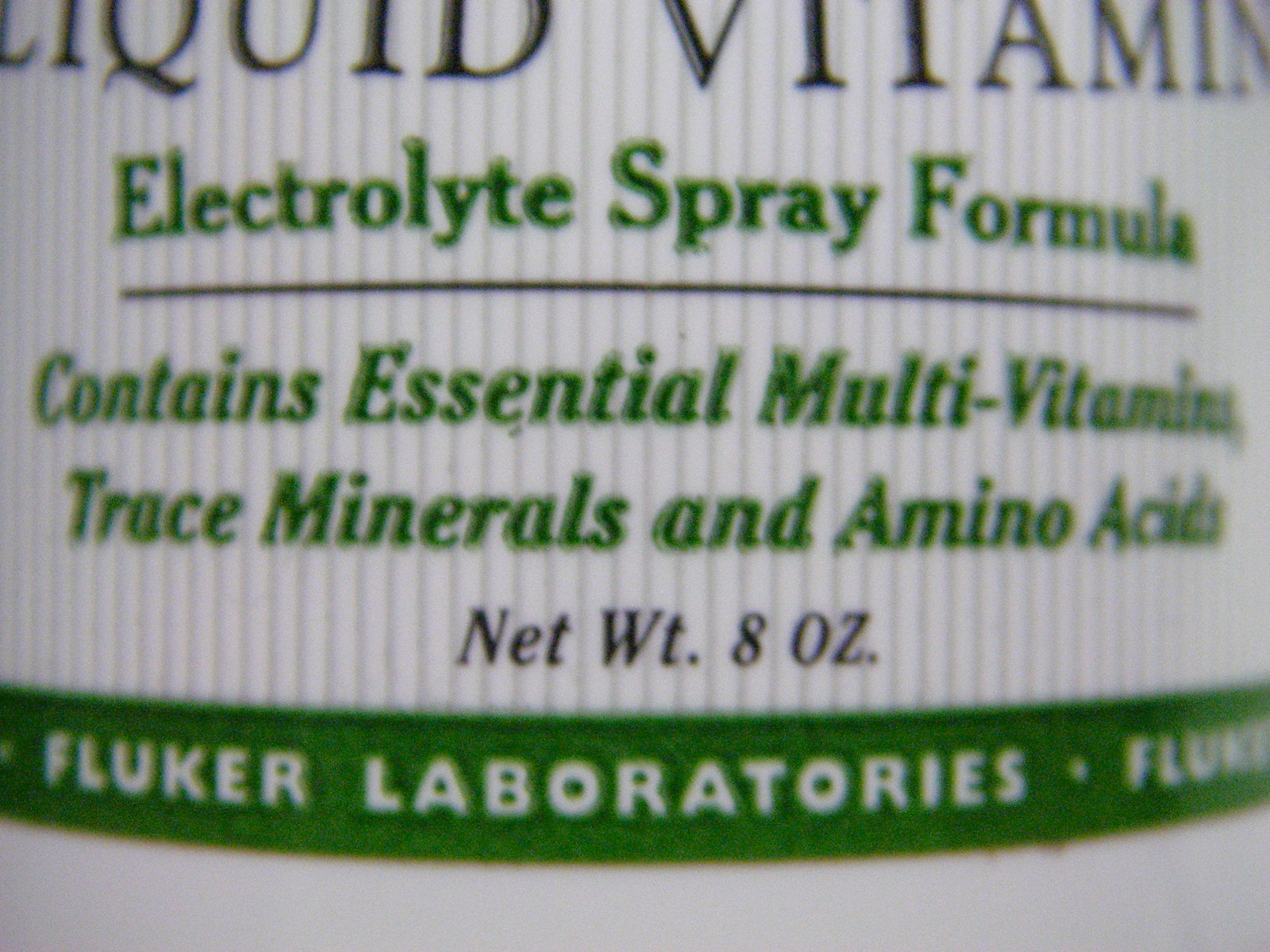The image is a detailed close-up of a label on a vitamin bottle. The label features a white background with silvery gray vertical lines running from top to bottom. At the top, in black capital letters, are the words "LIQUID VITAMIN." Beneath this, in green font, it reads "Electrolyte Spray Formula." Further down, still in green, it states "Contains essential multivitamins, trace minerals, and amino acids" in a slanted font. Below this, in black font, the label indicates the product's net weight of 8 ounces. At the bottom of the label, set against a green band, are the words "Faulkner Laboratories" in white font, which appears to repeat around the base of the bottle. The image solely focuses on the label, highlighting its design and text details.